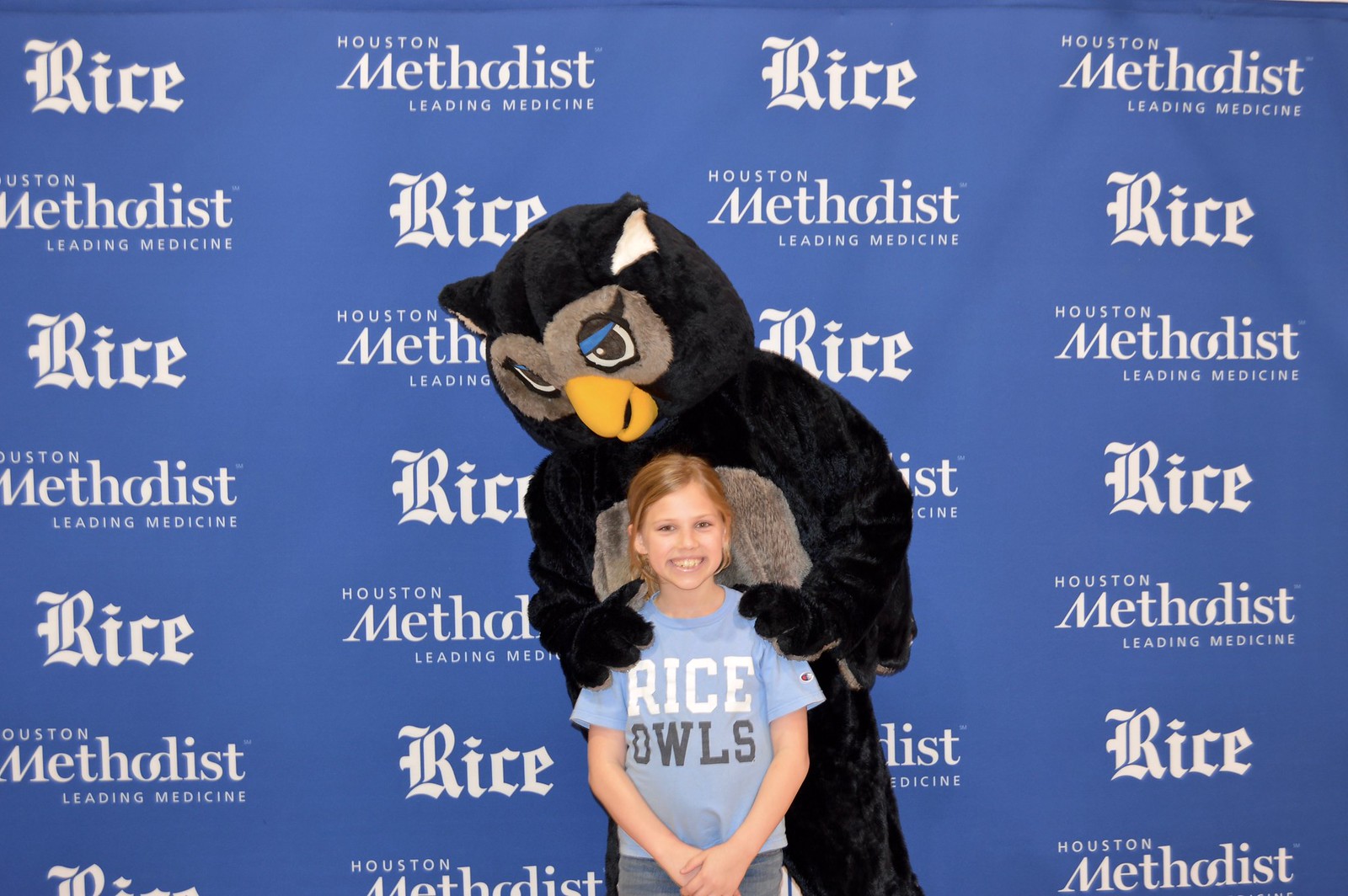In the photograph, a blonde little girl, around 10 years old, stands smiling in front of a blue backdrop featuring white text that alternates between "Houston Methodist Leading Medicine" and "Rice" arranged in four vertical columns. She wears a sky blue t-shirt emblazoned with "Rice Owls" in white lettering and has her arms relaxed in front of her. Behind her, a person dressed in a black owl mascot costume, accentuated with white ears, a yellow beak, and big round black eyes with blue eyelids, rests their hands gently on her shoulders. The owl, with a gray outline around its eyes, looks down at the girl, its head slightly tilted. The scene suggests the photo was possibly taken at a charity event or community gathering, with the backdrop displaying sponsors' names, reinforcing the event-like atmosphere.